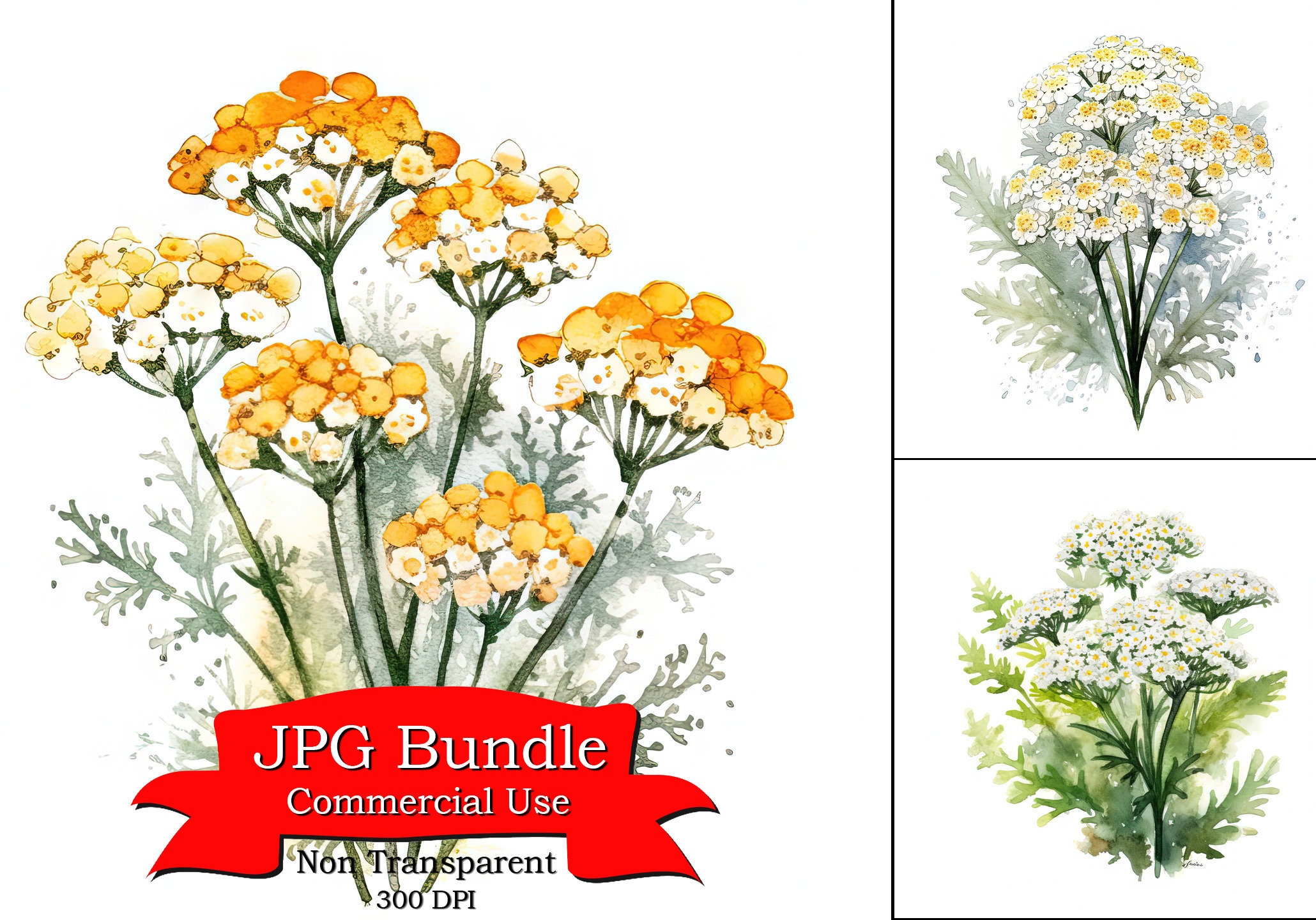This digital artwork mimics a watercolor style and showcases a prominent bundle of flowers positioned on the left-hand side. The main bundle is an elaborate arrangement of orange flowers, accompanied by greenery that appears somewhat reminiscent of chicken feet. Beneath this florid cluster, a red banner with white text reads "JPEG bundle commercial use," followed by "non-transparent 300 DPI." To the right of the primary bundle, there are additional options featuring similar floral designs but with varying treatments. One alternative bundle displays white petals with golden centers, possibly invoking the look of Queen Anne's Lace due to its flat-topped appearance. Another smaller bundle mirrors this design, consisting of white petals with gold centers accentuated by black specks, complemented by leaves that are broader and more filled out than those of the main arrangement.